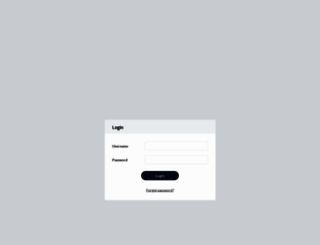**Descriptive Caption:**

The image marketing a business features a somewhat cluttered and out-of-focus composition, making details challenging to discern. At the top of the page, a white border spans across the image. In the top left corner, a stylized logo accompanies the barely readable text "Shoe Fun Media." In the top right corner, additional text options appear; however, they remain too blurry to interpret. 

Dominating the main portion of the image is a photograph depicting a city's skyline, with indistinct tall office buildings set against a clear blue sky peppered with a few clouds, suggesting a bright and pleasant day. On the lower right corner, there are elements that might be other office buildings or possibly trees, though these too are blurry.

On the right side of the image, a laptop computer with its screen turned on is visibly positioned. The laptop screen shows indistinct text and features four circular icons, each containing a photo of a person and a label with unreadable text.

Overlaying the image, the text reads: "Expose your content to new audiences, maximize reader engagement, and make money." Below this call-to-action is an orange button with the prompt, "Get Free Widget." Beneath the photograph, the text invites viewers to "join our native content discovery and advertising platform today."